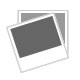The advertisement for Schwarzkopf Professional's Peptid Repair Rescue features a sleek, predominantly white background with accents of pink and red, reflecting the brand's color scheme. The Schwarzkopf Professional logo, along with a side profile silhouette, is prominently displayed at the top right. On the left side of the image, under the header "Your Old Favorite" within a gray border and white letters, are three containers of the previous product iteration with white bodies and red lids. The right side introduces "Your New Favorite" on a red banner with white letters, showcasing the updated product packaging: similarly shaped containers but with pink bodies and red lids. Above this visual transition is a bold red banner that reads "Peptid Repair Rescue," accompanied by prominent text stating "What's Changed?" Highlights of the new product, including "Skincare Inspired Ingredients, Premium Packaging, and New Technology," are also listed, emphasizing advancements from the old to the new version.